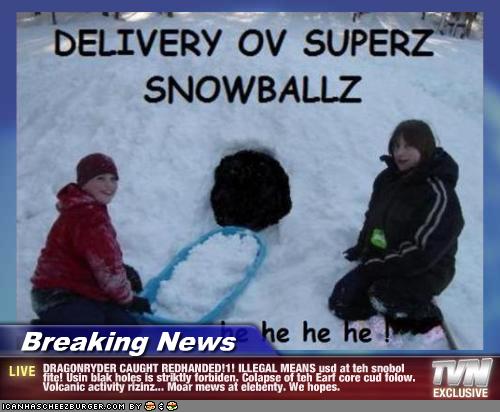The image is a screenshot from a TVN network broadcast, showing a winter scene with two kids dressed in snow gear, seemingly building an igloo or a snow fort. The boy on the left is holding a blue sled filled with snow, and there's a large black hole at the center, possibly part of their snow construction. At the top of the image, a caption reads "Delivery OV Supers Snowballs," with "snowballs" spelled with a "Z." Below the scene, overlapping banners display chaotic and misspelled text: a blue and white banner states "Breaking News," and a red banner beneath it reads "Live: Dragonrider caught red-handed. Illegal means used at the snowball site. Using black holes is strictly forbidden. Collapse of Earth's core could follow. Volcanic activity rising. More views at... We hope." Finally, at the very bottom, there's a humorous "I can has cheeseburger.com" line along with cheeseburger emojis.